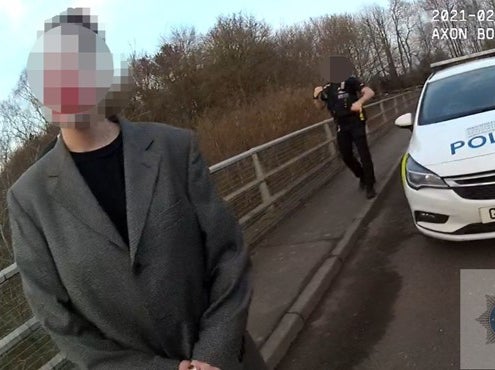This photograph captures a tense moment on a bridge during what appears to be a police encounter, potentially from a dash cam or a body cam. The scene is outdoors on a bridge, identifiable by the metal railing with wires running horizontally between the rails. The left half of the image prominently features a man wearing a gray jacket over a black shirt, although his face is blurred out. Trees can be seen in the background, adding depth to the scene. Walking towards this individual is a police officer dressed in a standard black police uniform, including black shoes and pants. The officer's face is also obscured and he appears to be holding something possibly a flashlight or his radio, with one hand close to his equipment. Just to the left of the officer is a white police cruiser, distinguishable by its blue lettering and the lights on top. The timestamp on the top right indicates the year 2021, month 02. The photograph captures a pivotal moment, with the officer approaching the individual, suggesting a law enforcement interaction taking place.